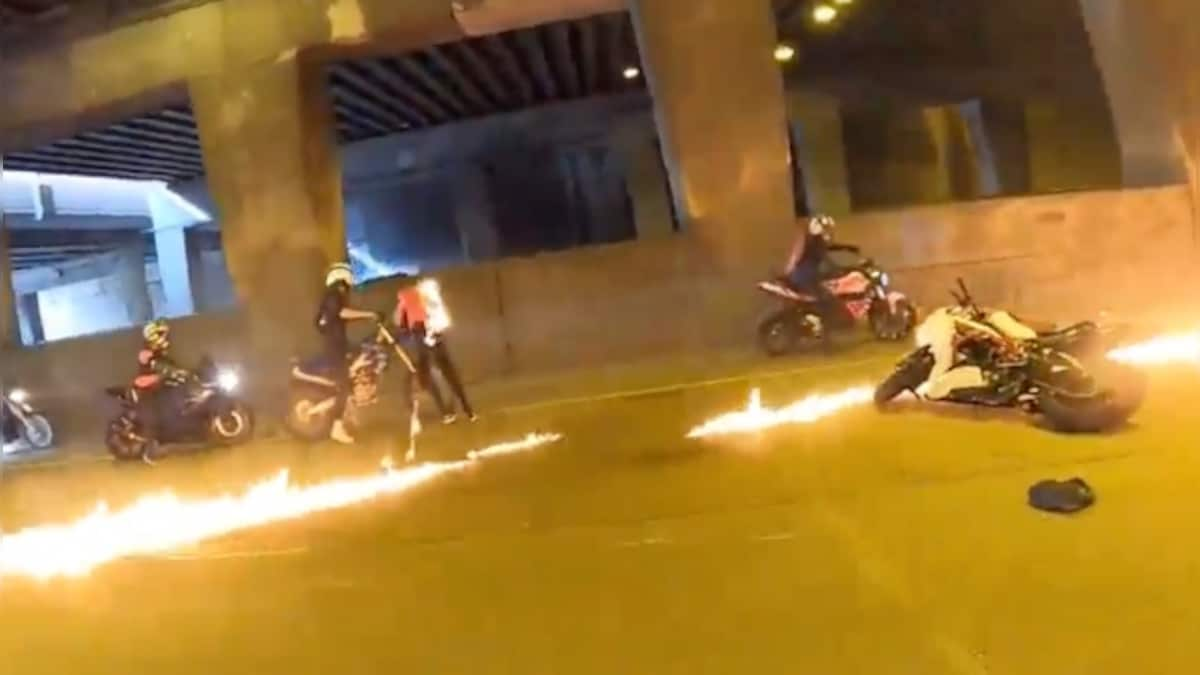In a dimly lit parking garage with concrete surroundings, the scene is illuminated primarily by the unsettling glow of flames scattered on the ground, supplemented by natural sunlight streaming in from the top left corner. The lighting casts a yellowish hue over everything. At the center of the chaos, five motorcycles are present. Four are upright, and one lies on its side near the right-hand middle of the image, surrounded by streaks of fire. The fallen motorcycle's front wheel is facing backward, with its back wheel towards the scene's center. 

All the motorcyclists are wearing white helmets and dark-colored jackets, suggesting they are together or part of a group. On the left side of the image, a person in a red shirt and black pants, carrying a glowing backpack, stands next to another individual leaning on a motorcycle. This person in red seems to be engaging with someone, possibly indicating some form of communication or concern regarding the events unfolding.

The motorcycles appear to be in various positions, with three grouped towards the left side and one on the right side, except for the scattered parts of the bike that fell over. The image conveys a tense moment, as the riders seem to be either reacting to or causing the dangerous situation with the flames, indicating a potentially critical or dramatic scenario.